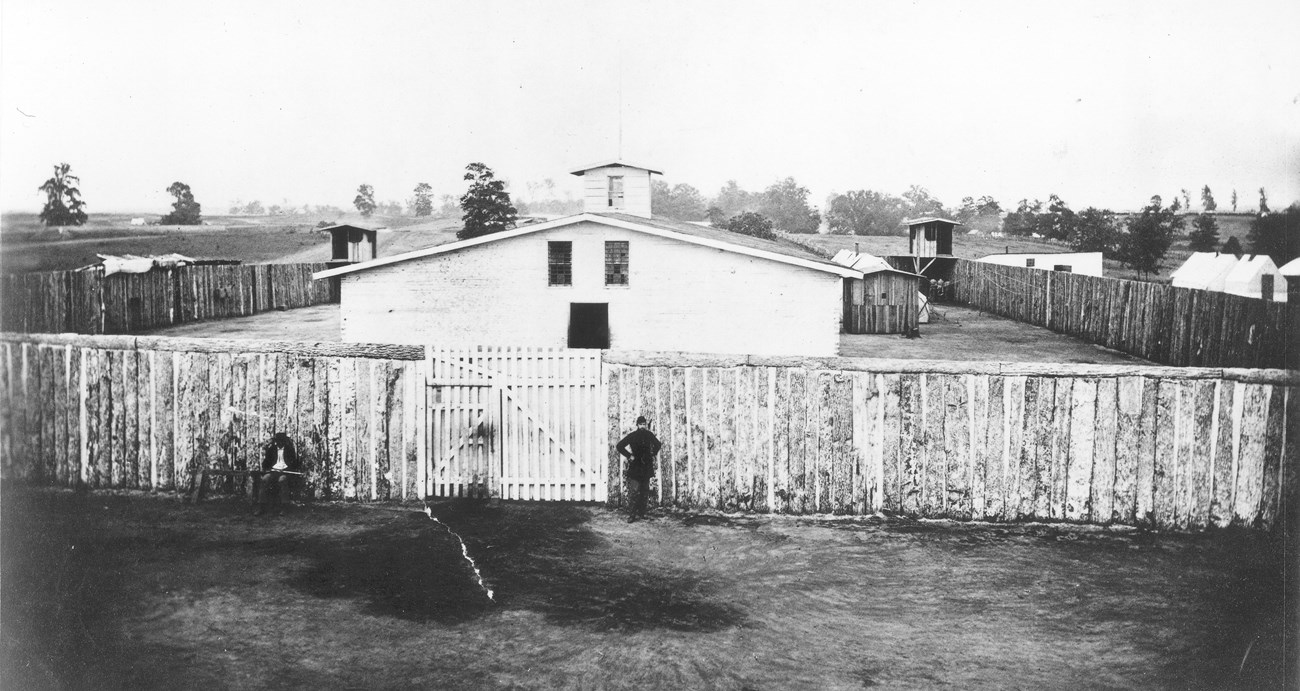This black-and-white photograph, likely taken on a hazy day, depicts a simple white farmhouse situated on flat terrain. The farmhouse, constructed from white brick and featuring two windows on its upper level and a large black door on its front, is surrounded by a sturdy wooden plank fence on all sides. A smaller white picket gate marks the entrance to the courtyard, where the main building contrasts with the landscape in its stark simplicity. In the immediate foreground, near the gate, stands a person dressed in black, while another figure sits on a bench to the left of the entrance. To the right of the farmhouse, a wooden shed adjoins the structure. The distant background reveals a row of scattered trees and what appears to be white tents, which might indicate a camping site or temporary dwellings. Additionally, there are hints of a raised guard post station at each corner of the enclosure, suggesting it could be a secure or monitored area.